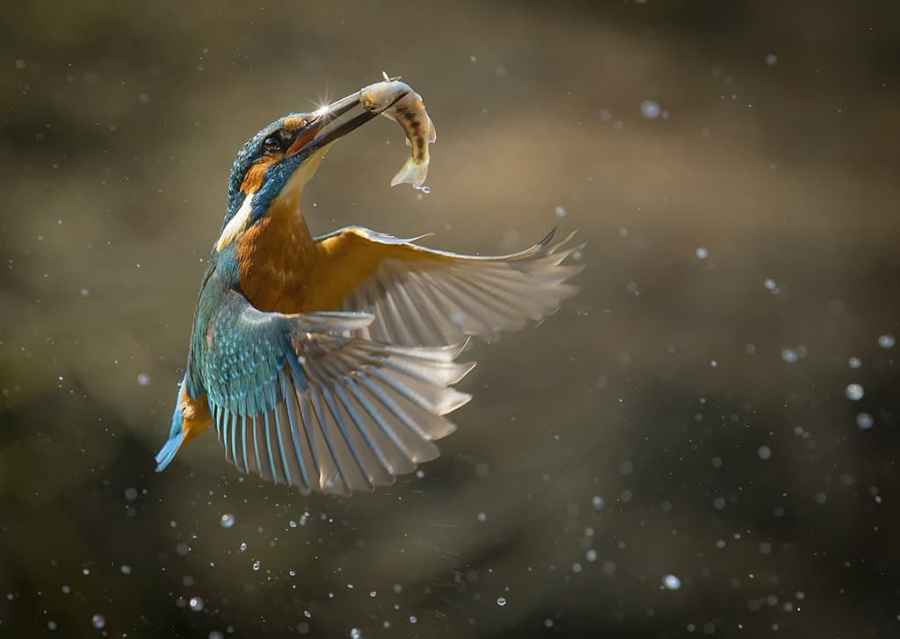This dramatic and expertly captured photograph showcases a vibrant kingfisher in mid-flight. The bird, which displays a striking array of colors, features orangish-yellow feathers on its chest and underbelly, transitioning to greenish-blue feathers on its wings, back, and tail. The greenish-blue hue extends up its neck towards its long, sharp beak, which is accentuated by a glistening reflection indicating bright daylight. The kingfisher has just emerged from a watery surface, with numerous water droplets suspended mid-air around it, providing a dynamic sense of action and motion. The kingfisher is clutching a small, brown fish with black dots along its side in its beak. The background of the photo is beautifully blurred into a soft brownish-grey, allowing the vivid colors of the bird and the sparkling water droplets to stand out prominently. The combination of fine details and the moment captured in mid-action marks the photograph as a breathtaking piece of wildlife photography.